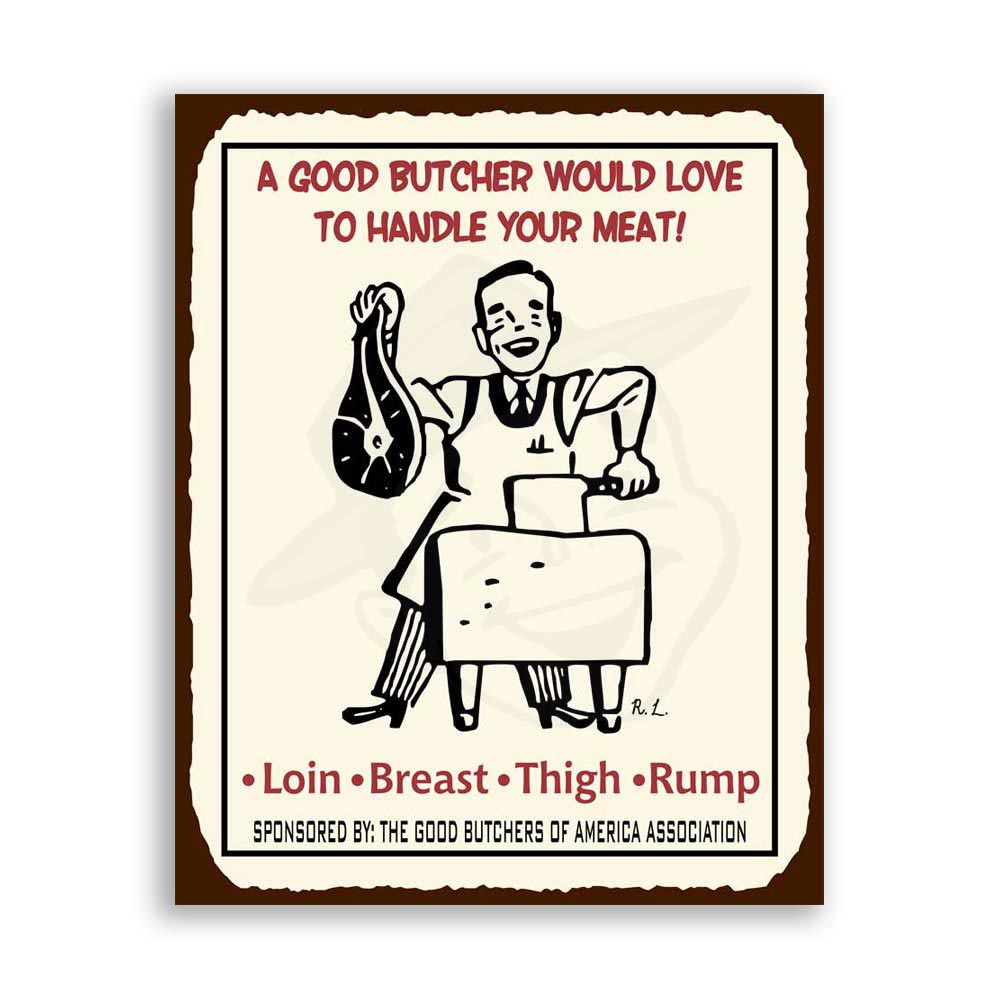This tall, rectangular poster features a playful and humorous design. The poster has a dark brown, hand-drawn-looking border that is thicker at the corners, creating a slightly uneven appearance. Against an off-white background, there's a bold black rectangle framing the content. At the top, in striking bold red letters, it reads, "A good butcher would love to handle your meat!" Below this, a black-and-white drawing showcases a cheerful butcher, adorned in a butcher's vest and tie. In his right hand, he holds a slice of beef, while his left brandishes a butcher's knife, all in front of a butcher's table. The figure is completed with him wearing boots. A faint gray shadow extends to the left and underneath the poster, adding depth to the image. Notably, there is also a subtle silhouette of a smiling cow behind the butcher. The bottom of the poster lists, "loin, breast, thigh, rump" in bold red letters, with an emblem indicating the sponsorship by the Good Butchers of America Association. This poster, blending vintage-style art and humor, could make a charming and amusing addition to a kitchen or butcher shop.